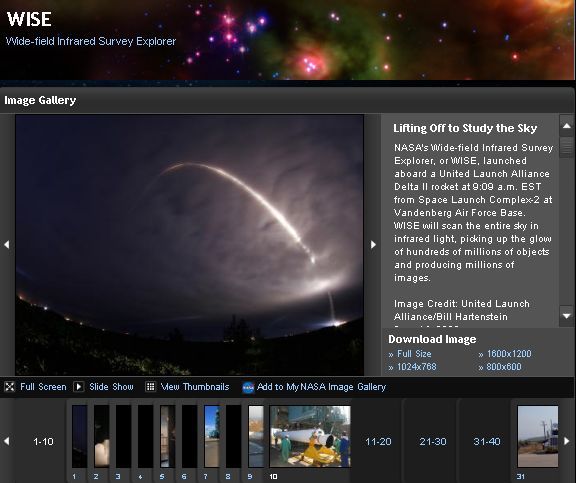This image is a screenshot of a program titled "Wide Field Infrared Survey Explorer" (WISE). In the upper left-hand corner, the word "WISE" is prominently displayed in white capital letters, with the full name "Wide Field Infrared Survey Explorer" written in blue beneath it. 

Across the top, there is a vibrant banner image depicting a colorful rendering of outer space, possibly a bright galaxy. The image is scattered with numerous star-like dots and varying shades of color representing galaxies, featuring hues of pink, blue, purple, green, orange, and black.

Beneath this banner, the background transitions to gray, housing various menu options, images, and text. At the top of this section, the heading "Image Gallery" is displayed.

The main focus of the image is a photograph showing a cloudy night sky with an arc of white light, suggesting a fisheye lens was used to capture this expansive view. To the right of this photograph, white text provides detailed information about the image:

"Lifting off to study the sky, NASA's Wide Field Infrared Survey Explorer (WISE) launched aboard a United Launch Alliance Delta II rocket at 9:09 a.m. Eastern Standard Time from Space Launch Complex 2 at Vandenberg Air Force Base. WISE will scan the entire sky in infrared light, picking up the glow of hundreds of millions of objects and producing millions of images."

This detailed caption captures the essence and context of the WISE program and its mission to explore the universe in infrared light.